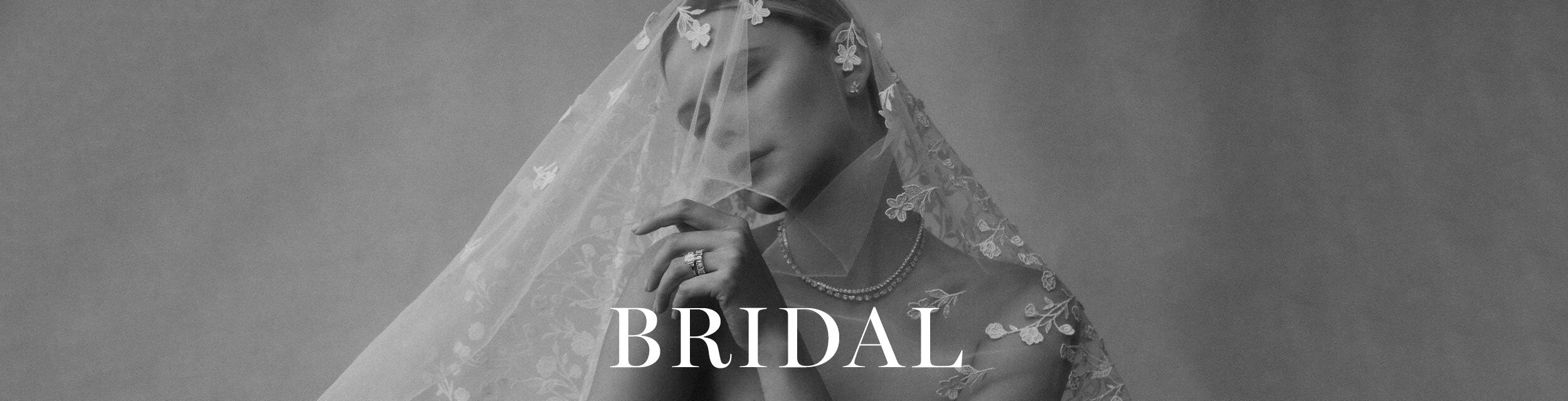The photograph is a monochromatic advertisement for a bridal company, presented in a long, wide rectangular format. It features a model resembling a bride, depicted in black and white, with the word "BRIDAL" prominently displayed in all-capital white serif font at the bottom center. The model is adorned in a Chantilly-style veil with intricate floral embroidery, which drapes over her face and down her back. Her head is gently tilted to the left in a contemplative pose. She wears a pearl necklace and an engagement ring on her raised left hand, which is positioned near her face as if she's daydreaming or admiring the ring. Her hair is neatly pulled back, adding to the elegant simplicity of the image. The background remains a simple gray, drawing attention to the detailed textures and elements of the bride's attire.